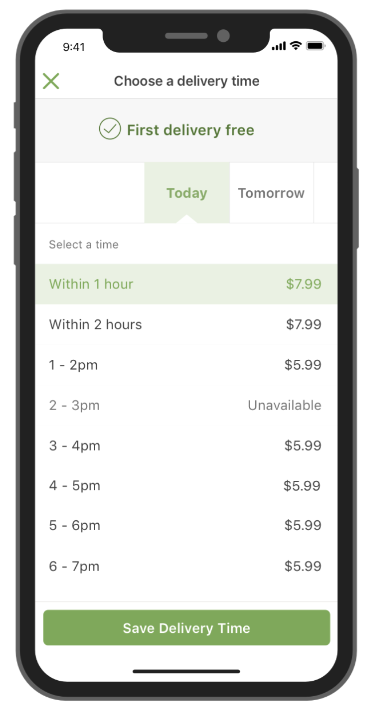The image is a clear, detailed screenshot of a mobile phone, showcasing both the device itself and its display. On the left side (top left edge) of the phone, the volume buttons are visible, while the right side features the power button. The phone's screen displays an app interface with a prominent section titled "Choose a Delivery Time." Directly beneath this title, there is a label "First delivery free" with a green checkmark beside it, indicating a promotional offer.

Below the promotional label, there are two options: "Today" and "Tomorrow," with "Today" highlighted in green, suggesting it is the selected option. Further down, there is a list of delivery time slots and their associated costs. The options include:

- "Within one hour" highlighted in green with a cost of $7.99
- "Within two hours" at $7.99
- "Between 1:00 PM - 2:00 PM" at $5.99
- "2:00 PM - 3:00 PM" grayed out, indicating it's unavailable
- "3:00 PM - 4:00 PM" at $5.99
- "4:00 PM - 5:00 PM" at $5.99
- "5:00 PM - 6:00 PM" at $5.99
- "6:00 PM - 7:00 PM" at $5.99

At the bottom of the screen, there is a green "Receive Delivery" button. The app's interface is set against a clean white background.

In the top right corner of the phone's display, the battery icon is visible, while the top left corner displays the time, 9:41. Positioned between the time and the battery icon at the top is the phone's front camera.